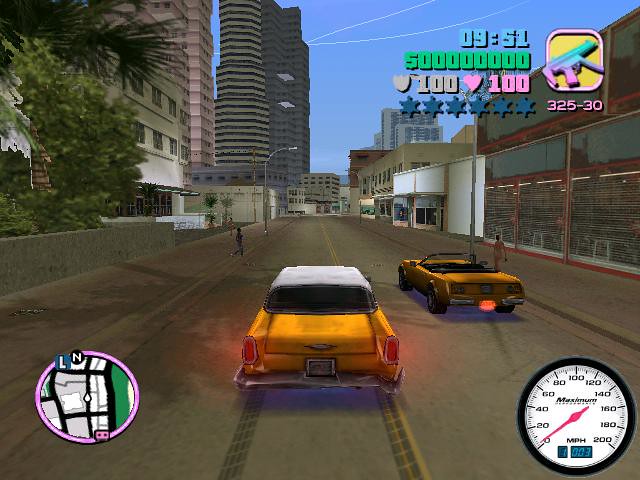This screenshot from the video game "GTA Vice City" features a vivid scene depicting the player driving a vintage yellow vehicle, reminiscent of the 1960s or 1980s. The car is presently halted, evidenced by the illuminated brake lights and the tread marks left on the road. The in-game time displayed is 9:51, and notable HUD details include the player's status: no available money, but full health (100%) and full armor (100%). The player is armed, with a weapon holding a total of 325 rounds, divided into magazines of 30 cartridges each. The scene is set near a beachfront location, as indicated by the map situated in the lower left corner of the screen. On the lower right side, a speedometer shows the vehicle's speed at a mere 3 miles per hour.